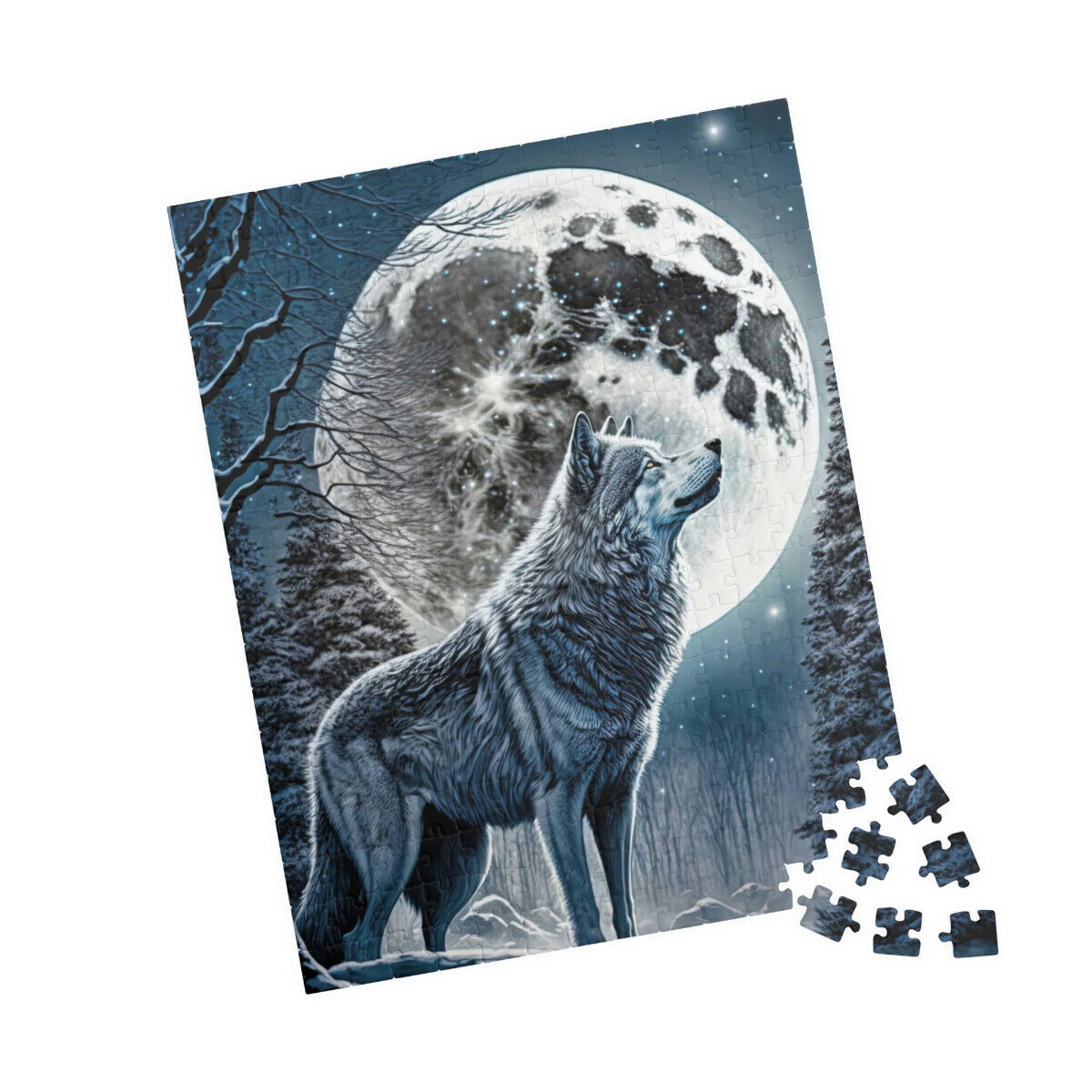This image showcases a nearly completed rectangular jigsaw puzzle featuring a detailed, color portrait of a gray wolf with a white muzzle and ears standing straight up. The wolf is positioned in profile, gazing to the right, set against a wintry outdoor landscape. The background is dominated by an enormous, white-gray full moon that occupies a significant portion of the scene, illuminating the night sky sprinkled with stars. The setting includes snow-covered evergreen trees flanking either side of the wolf, and bare tree branches in the foreground further enhancing the wintry atmosphere. The puzzle is tilted back at an angle of about 10-15 degrees, and although most of the puzzle appears seamlessly assembled, the bottom right corner features six disconnected pieces spread out, showcasing the nearly finished state of the puzzle. The overall color palette is composed of serene grays, blues, whites, and blacks, accentuating the tranquil yet majestic wilderness scene.